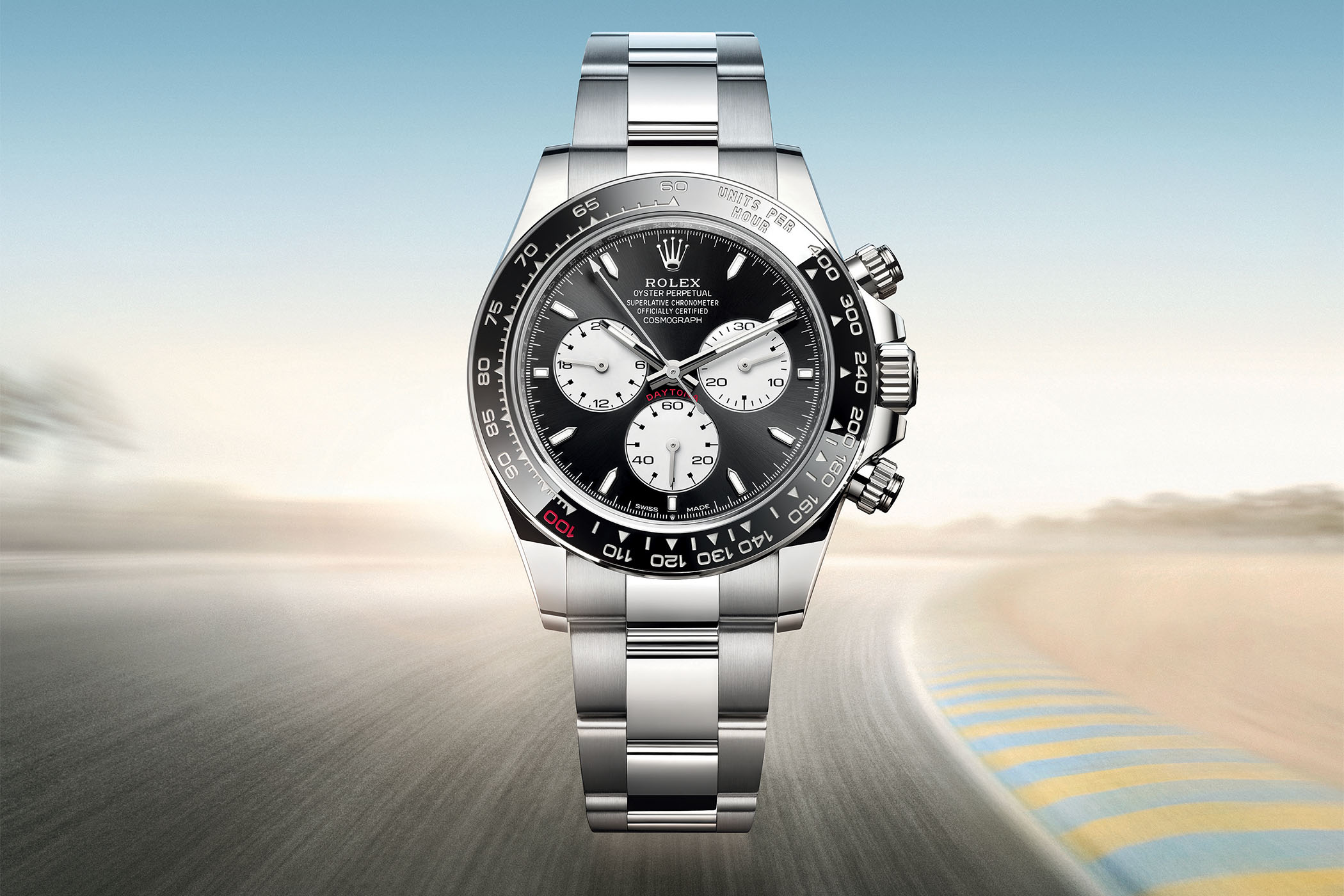The image is a highly realistic, colored photograph of a Rolex watch, likely created for advertising purposes. The watch, prominently featured in the foreground, has a sleek silver band and a striking black face adorned with white details. Central to its design are three smaller sub-dials and the Rolex logo, along with the word "Daytona" elegantly inscribed on the face. The timepiece has black and white hour and minute hands, along with a white second hand ending in a small arrow. The outer edge of the watch face is bordered with numbers ascending to 400, labeled "units per hour." The background, which appears digitally rendered or edited, depicts a blurry racetrack under a blue sky, suggesting speed and precision, enhancing the advertisement's dynamic appeal.